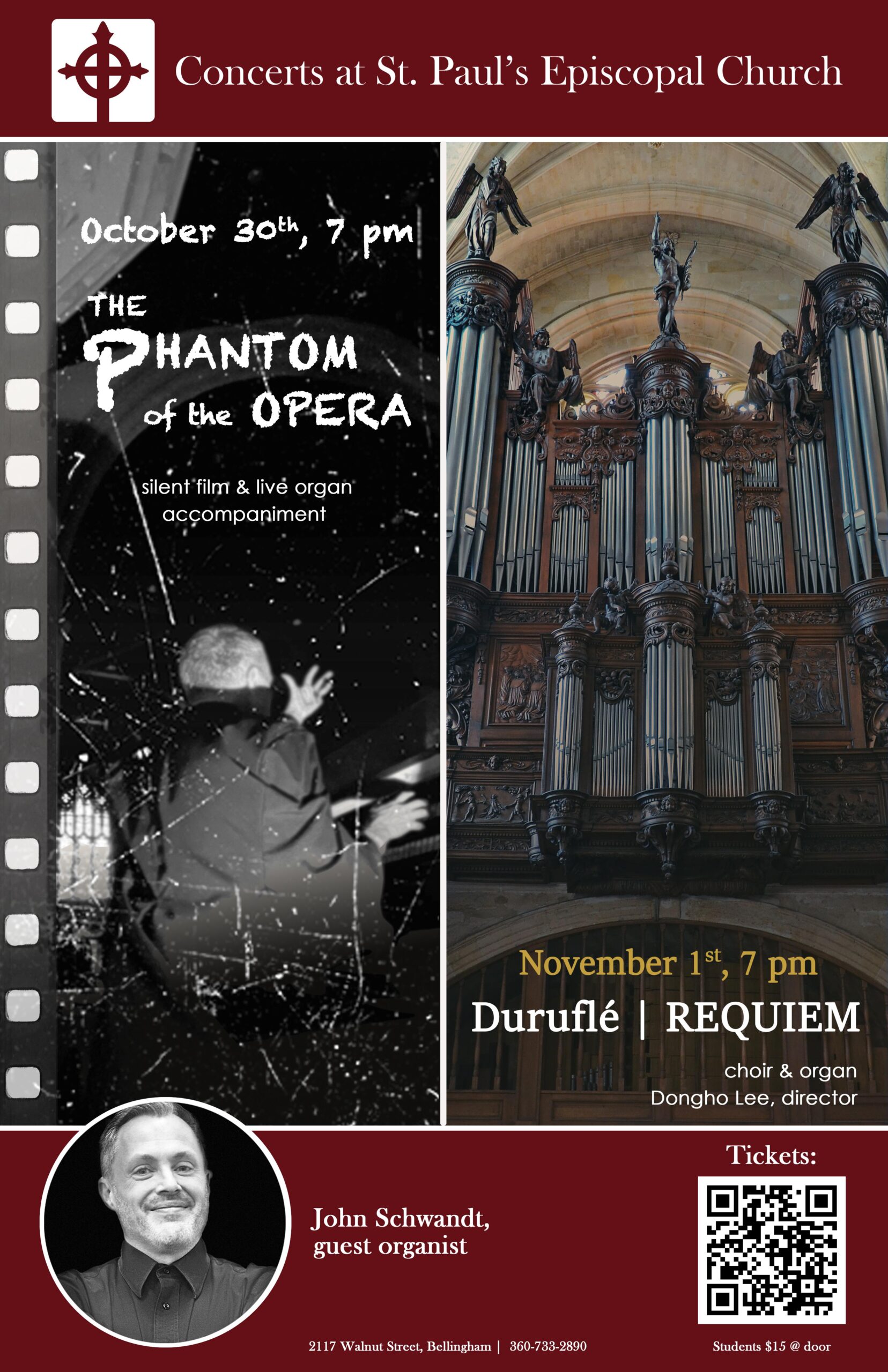This image appears to be the cover of a flyer or a book. At the top, there is a prominent red banner featuring a cross encircled by a ring, symbolic of St. Paul's Episcopal Church. On the upper left-hand side, there is a white square that encases this emblem. Below the banner, in bold white lettering, the text reads "Concerts at St. Paul's Episcopal Church." The main part of the flyer contains two distinct images. The image on the left is a scene from the "Phantom of the Opera," depicting an actor with his back turned to the camera. The right-hand side showcases an interior view of St. Paul's Episcopal Church, highlighting its architectural beauty and likely setting for the concerts.